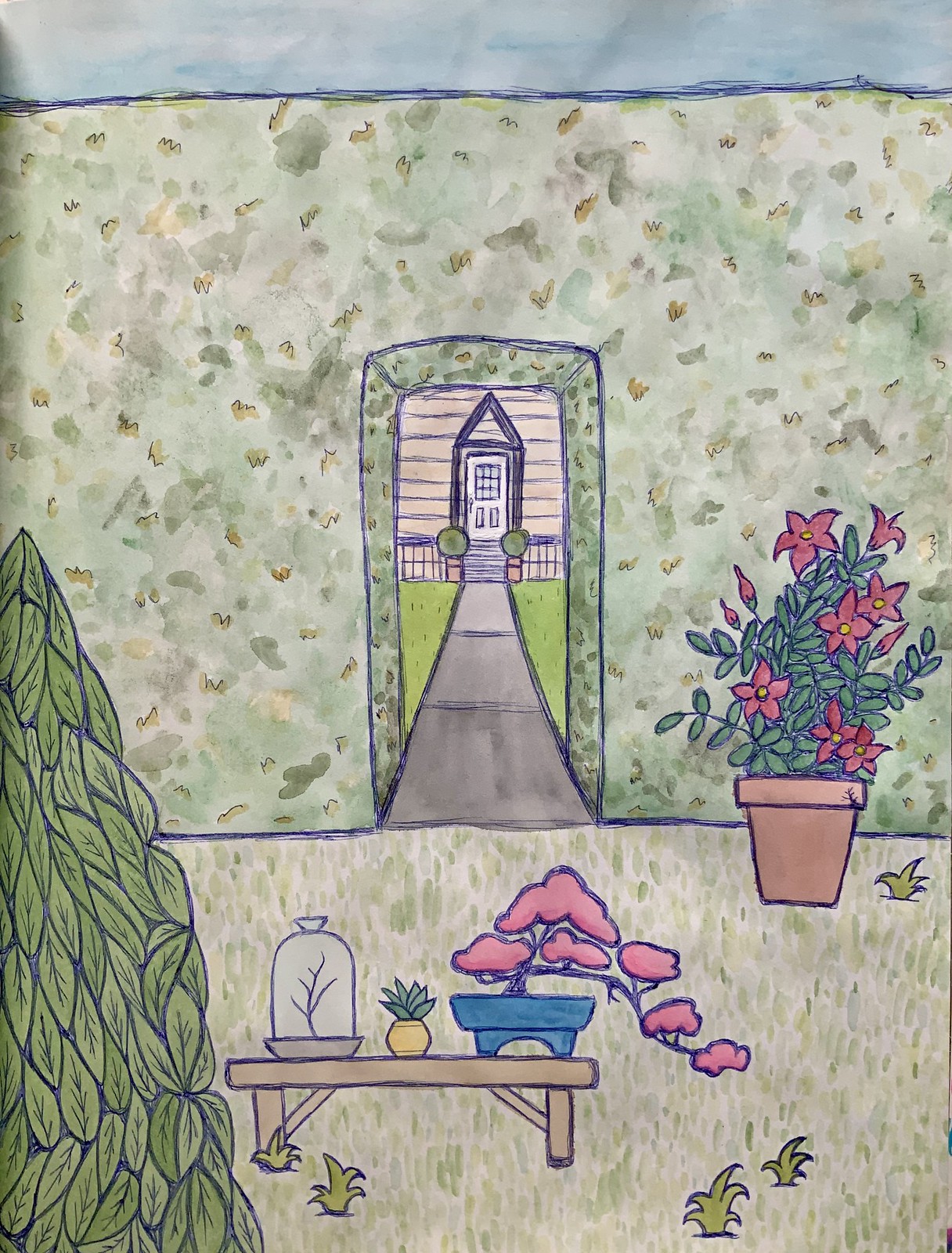This animated illustration showcases the interior of a room with a doorway leading to an exterior scene. In the bottom-left corner, there is a tree-shaped green house plant. Positioned in front of the plant, there is a light brown bench adorned with a yellow vase containing green leaves. To the right of this setup, a blue vase holding purple tree branches and pink leaves is prominently displayed. Adjacent to this, on the left, is a clear jar with a single tree branch. The floor is primarily white with subtle, faded green streaks running through it. Additionally, on the right side of the image, another house plant with pink flowers in a brown vase is visible. The walls above are speckled with gray, green, and brown. Through the doorway, a gray pathway leads to what appears to be the entrance of another house, with fields of grass flanking the path on both the left and right sides.